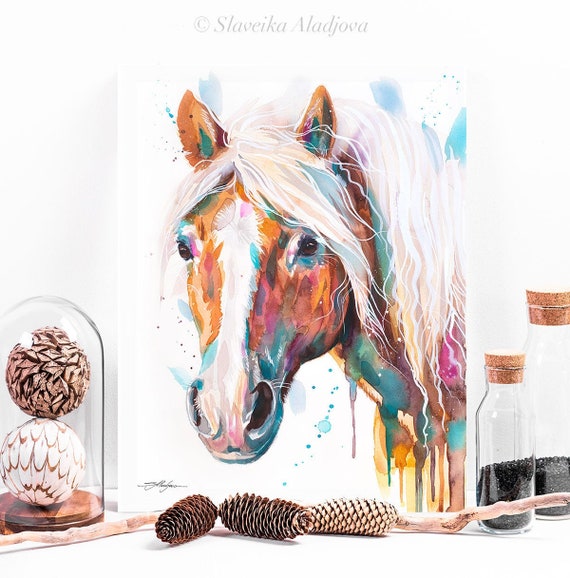This image features a rectangular watercolor painting of a horse's head against a white background, signed at the top in small gray text: "Copyright Slavica Alejova." The horse, facing forward, showcases a blend of vibrant colors: its white mane is streaked with orange and pink, interspersed with drips and splashes of blue, green, and yellow. The horse’s predominantly brown face is marked by a white stripe down the center, and its ears, tinged with orangish-brown and green, peek through the scraggly, wiggly mane. The head and neck are adorned with shades of brown, red, blue, and green, creating a dynamic, multi-colored effect, accented by paint splatters around the canvas.

In front of the painting, there are three brown pine cones and a stick devoid of leaves. To the right, two tall, rectangular glass jars with tan cork tops contain black seeds or beads. On the left, a large glass container holds two decorative balls; one is white with brown lines while the other is brown with patterns reminiscent of leaves. The simplicity of the white background accentuates the vibrancy of the horse painting and the earthy tones of the objects below.